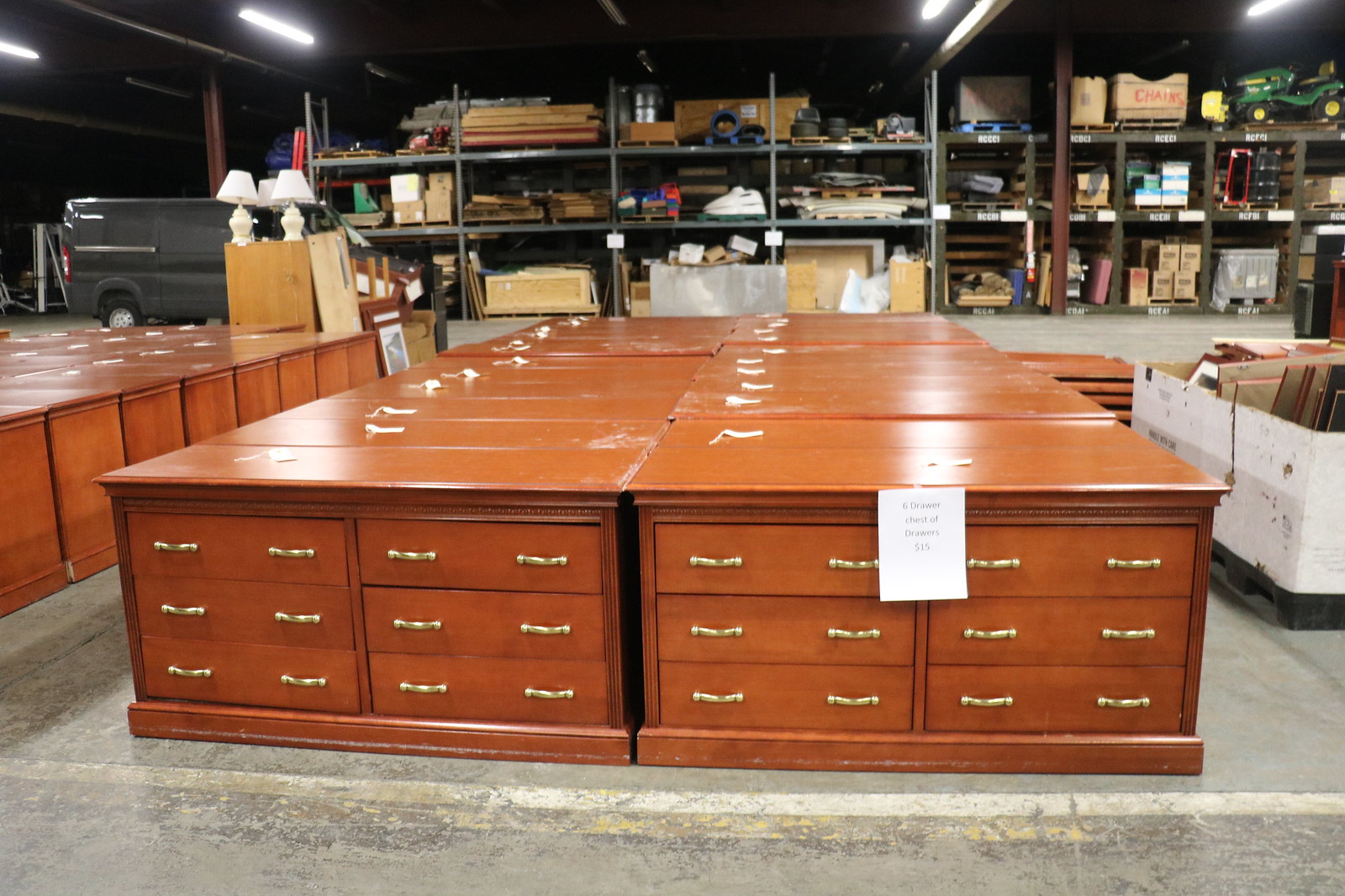The image depicts a spacious warehouse with a faded gray concrete floor, bisected by a white line. Central to the scene are two prominent rows of several wooden chests of drawers, all identical, with an additional similar row partially visible to the left. Each chest of drawers is made of rich red oak brown wood and contains six drawers, arranged in two rows of three. The drawers are accented by two vertical brass handles each, simple yet elegant. On top of each chest is a white paper tag, and the front desk in the right row has a paper with indistinct black text affixed to it. In the background, high-rise shelving spans three levels and is stocked with various items like boxes, wood, and construction materials. To the left, a grey cargo van is partially visible, while to the right, a large white box possibly filled with particle board stands out. Additionally, there's a box on the far left row containing white lamps with matching white shades.